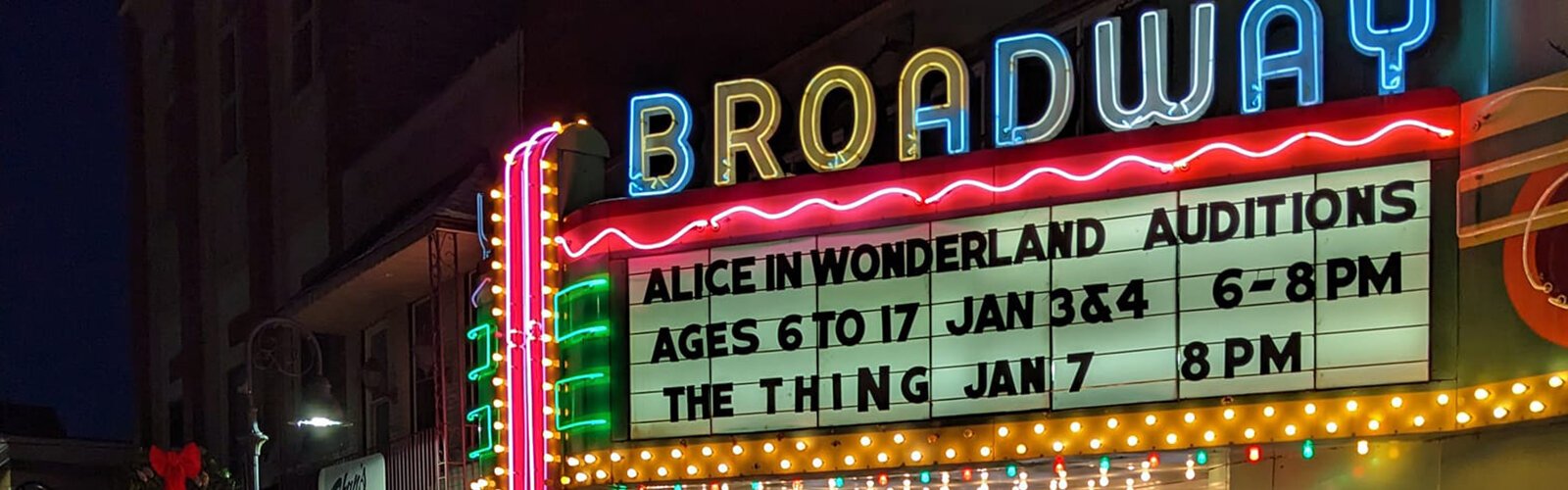In the photograph, there's a prominent movie theater marquee featuring a vibrant neon sign that reads "Broadway" at the top. The word "Broadway" is predominantly blue with yellow highlights; specifically, the letters R and O are entirely yellow while the A is mostly yellow. Directly beneath this, the billboard displays the text "Alice in Wonderland Auditions ages 6 to 17 January 3rd and 4th 6 to 8 p.m." and "The Thing January 7th 8 p.m." The sign is adorned with additional neon elements, including red squiggly lines, red straight lines, and a green three-quarters circle on the sides, while staggered yellow and white light bulbs line the bottom. The scene is set at night, as indicated by the dark sky and the streetlamp visible to the left of the sign, casting a glow that enhances the colorful radiance of the neon lights.